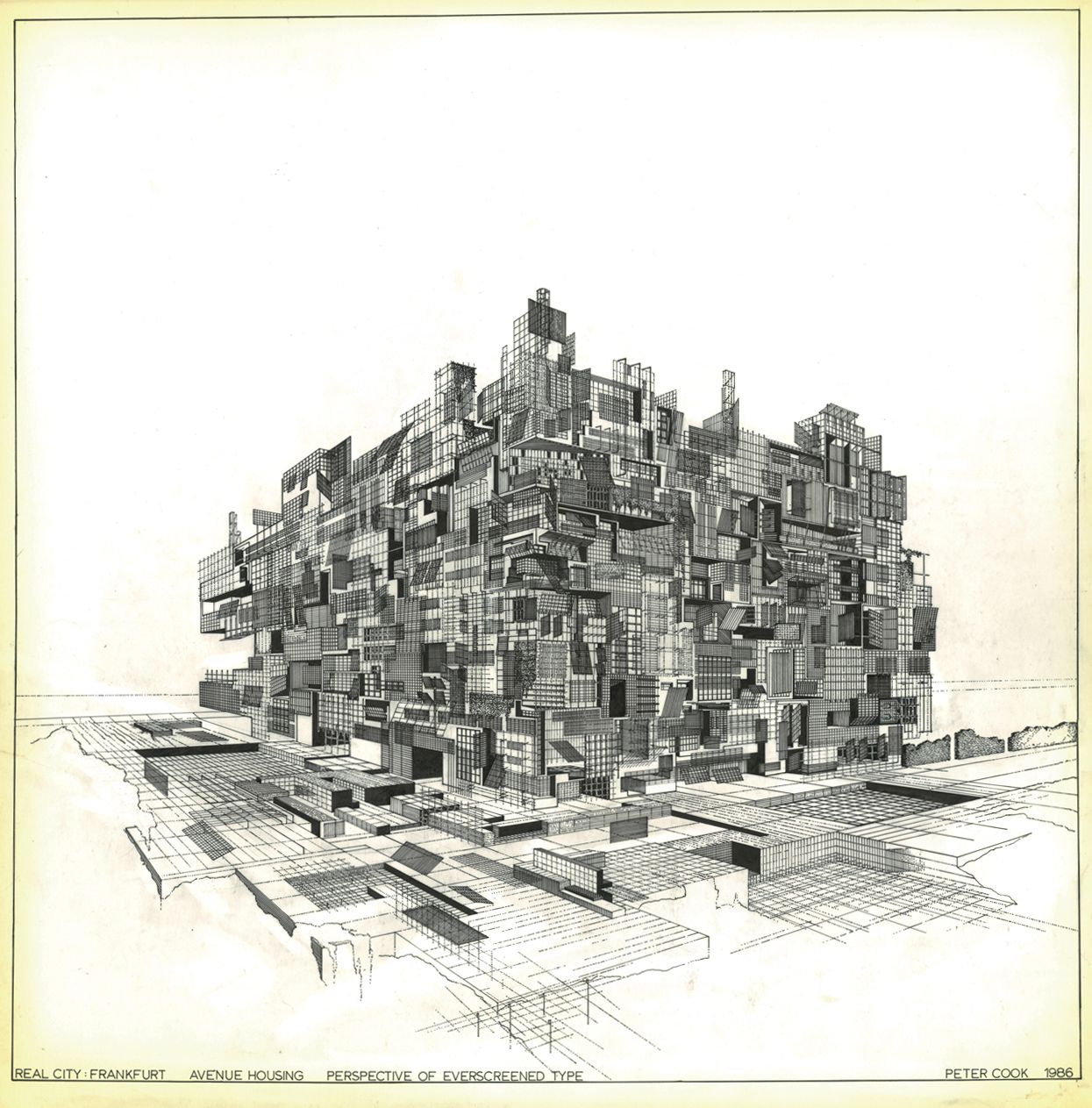This black-and-white sketch, an architectural draft by Peter Cook from 1986, is a detailed representation titled "Real City Frankfurt Avenue Housing Perspective of Eversgreen Type." The artwork features an intricate assembly of squares, rectangles, and polygons that interlock and stack to create a highly geometric and slightly abstract depiction of a building. The building design is composed primarily of cube-like forms and blocks, with discernible lines and window patterns. The page itself shows signs of wear, particularly yellowing at the edges, lending a vintage character to the sketch. The overall composition appears somewhat futuristic, with the ground plane also covered in crisscrossing squares and rectangles, reinforcing the complex and modernistic aesthetic of the piece.